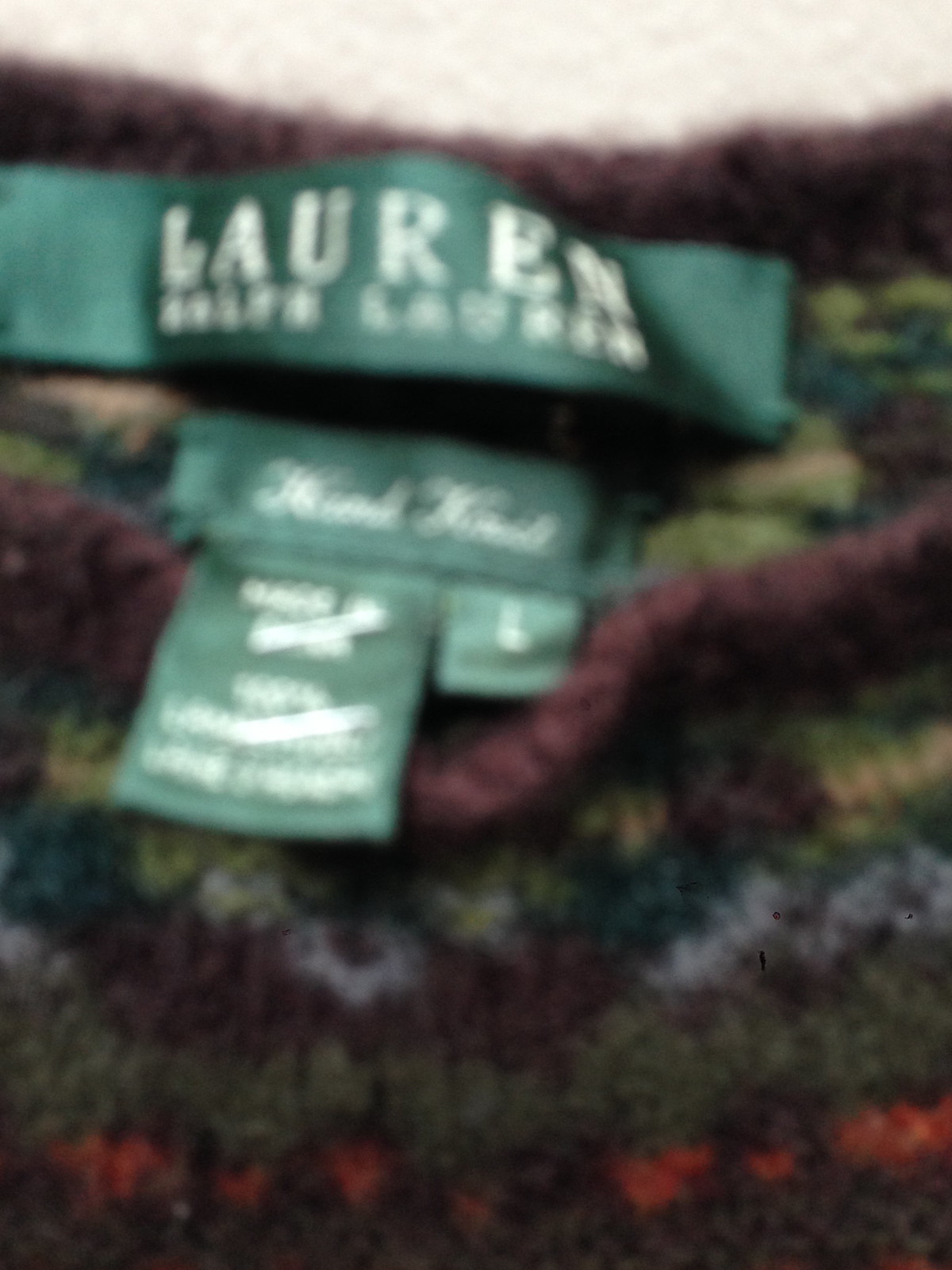A close-up, slightly blurred photograph captures the intricate details of a vibrant knitted sweater. The front and center of the image feature several dark green satin tags with white text, though much of the writing is hard to decipher due to the blur. The largest tag prominently reads "Lauren Ralph Lauren," while smaller tags beneath it likely detail washing instructions and fabric content, with one indicating the size as "LARGE."

The sweater itself showcases an array of colors woven into a zigzag stripe pattern, incorporating hues of lime green, blue, dark green, purple, violet, brown, and orange. On closer inspection, the upper section of the sweater includes a round neckline in a cranberry color, with other areas reflecting colors like olive green, gray, and burnt orange. The texture appears somewhat loose-knit, adding to the intricate, multicolored design. The top edge of the image reveals part of a white carpet, suggesting the photograph may have been taken in a domestic setting.